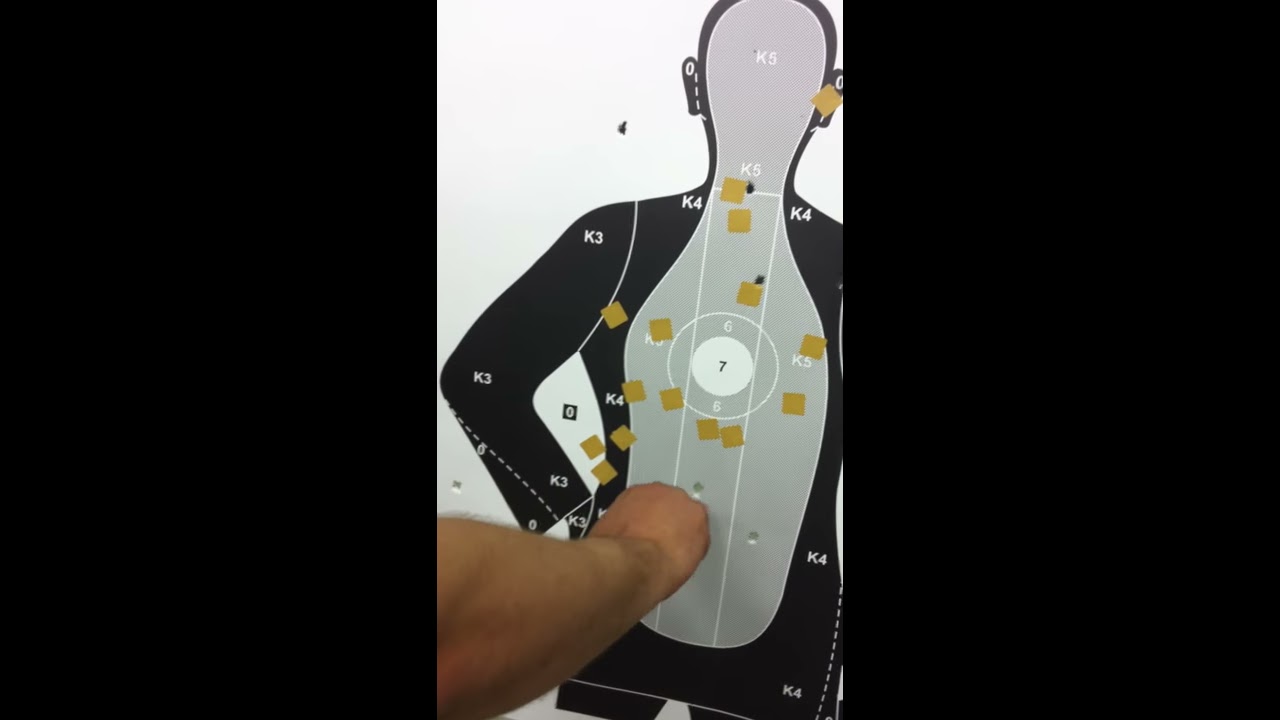The image depicts a human-shaped target at a firing range, framed by black rectangles on the left and right sides. Central to the image is a silhouetted target with a light-skinned man's arm extending from the left, his closed fist positioned as if punching or reaching into the target's midsection. The target itself, designed for firearms practice, features a gray and white color scheme with defined circular zones. The head, shoulders, arms, and torso are marked with labels such as K3, K4, K5, 6, and 7, and there are numerous gold squares indicating where bullets have struck. The chest area includes thin white vertical stripes and a prominent white circle surrounded by a gray circle with another smaller white circle in the center. This arrangement resembles a concentric target with clear demarcations for aiming and shot assessment.